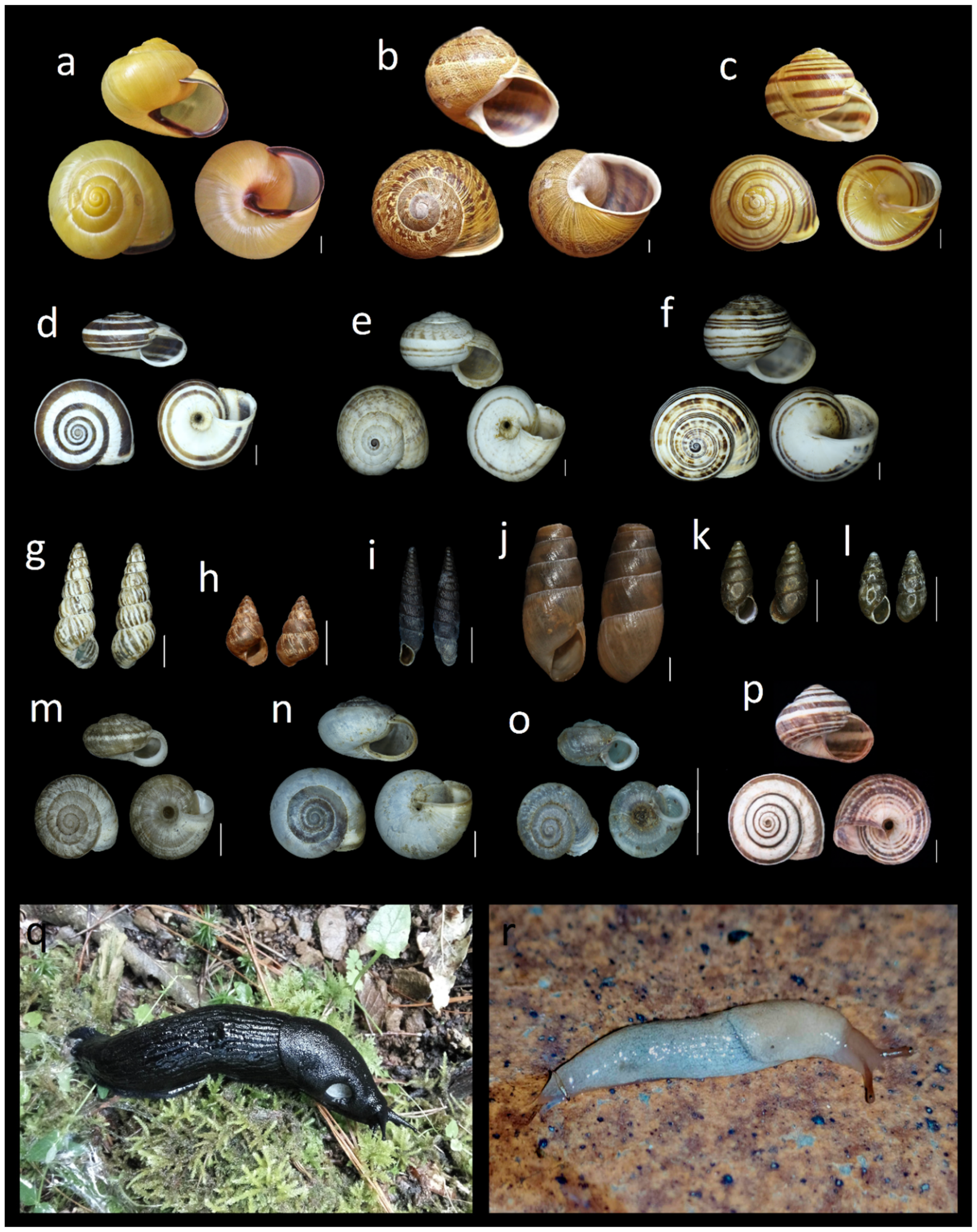The image is a detailed and methodically labeled illustration and photograph showcasing various types of snails and snail shells. At the bottom, there are two distinct photographs of shell-less snails. On the left, within a section labeled 'Q,' there is a dark black snail resting amidst green grass and sticks, resembling a natural habitat with vegetation. In the bottom right, within a section labeled 'R,' a translucent white snail is seen perched on a brown countertop, creating a stark contrast with its surroundings. Above these photographs, the image presents an extensive array of snail shells, arranged in four rows and labeled from A to P. Each shell exhibits unique designs and colors. The first row (A-C) features shells with swirled patterns in yellow and brown hues. The second row (D-F) continues the swirled motif but emphasizes white and brown colors. The third row (G-L) showcases more distinct, arrow-head or pinpoint styles with variations in white, black, and brown tones. The final row (M-P) returns to dulled circular swirled patterns, displaying grayish blue and reddish-white combinations. All shell images are set against a dark black background, enhancing their detailed textures and designs. This comprehensive visual display appears well-suited for use in a textbook or nature identification guide, providing clear and precise depictions of both the snails and their shells.